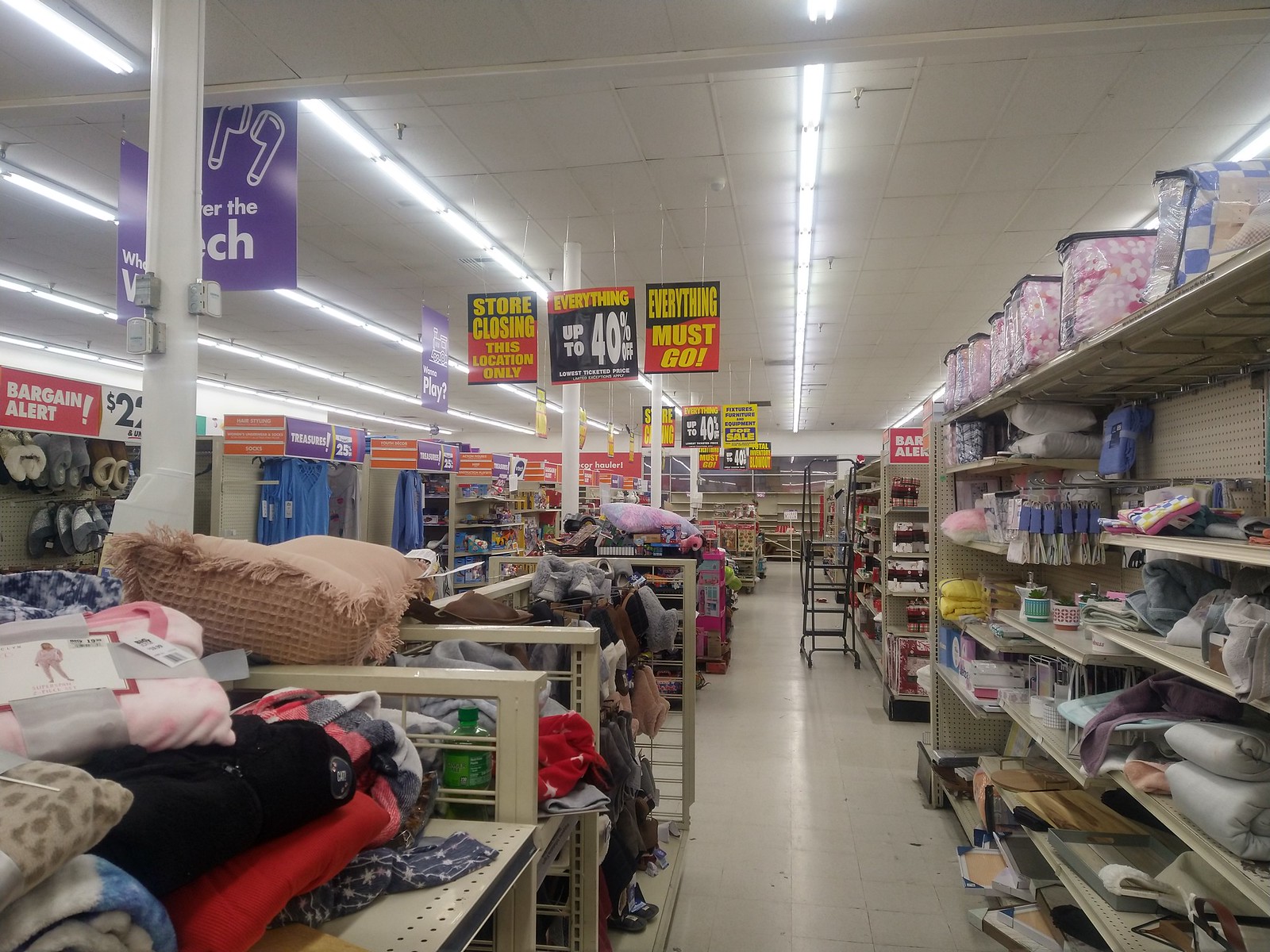This photograph depicts the inside of a large department or home goods store, reminiscent of a Walmart, Target, or similar retailer. The store is brightly lit with long, continuous fluorescent lights extending to the far end of the store from the white-paneled ceiling. The glossy white tile floor reflects the light, enhancing the store's brightness. Signs hanging from the ceiling prominently announce a "Store Closing" sale exclusive to this location, with discounts of up to 40% off on everything.

On the right side of the image, long shelves stretch down the aisle, stocked with a variety of household items including blankets, sleeping bags, and possibly soap dispensers and towels. Some shelves are cluttered with piles of clothes, contributing to a slightly messy appearance. In the foreground on the left, there are shorter shelves and racks, with items like women's pajamas, assorted blankets, pillows, and soft objects displayed. Further back on the left side, similar racks continue, showcasing more clothing and some footwear items, like slippers and clogs.

A striking "Bargain Alert" sign with a "$2" mark is visible on the left side. A column with three gray panels reaches up to the ceiling toward the back, potentially housing an intercom system. Throughout the scene, it is apparent that the store is in the final stages of liquidation, with products strewn and disorganized, symbolizing the urgency and finality of the "everything must go" sale.